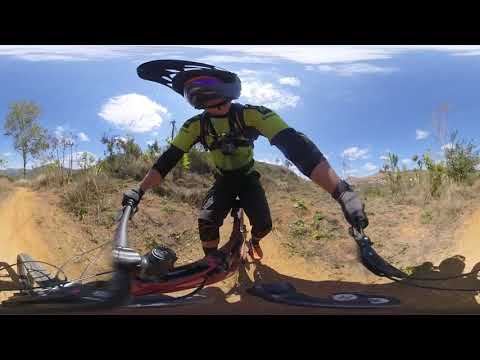In this dynamic and heavily edited image, we see a man clad in a light yellow cycling uniform with black accents, including armpads and gloves. He sports a black helmet adorned with purple goggles and rides a mountain bike along a dirt path. The perspective seems to be from the handlebars looking up at him, adding to the action shot feel. The background features a hilly, desert-like landscape with sparse greenery such as bushes, trees, and even some cactuses. The sky above is mostly blue with scattered white clouds, indicating a bright and sunny day. The scene is framed with black borders at the top and bottom, emphasizing the rugged outdoor setting. The rider appears centrally positioned in the image, actively navigating the sandy terrain, giving a sense of movement and adventure.